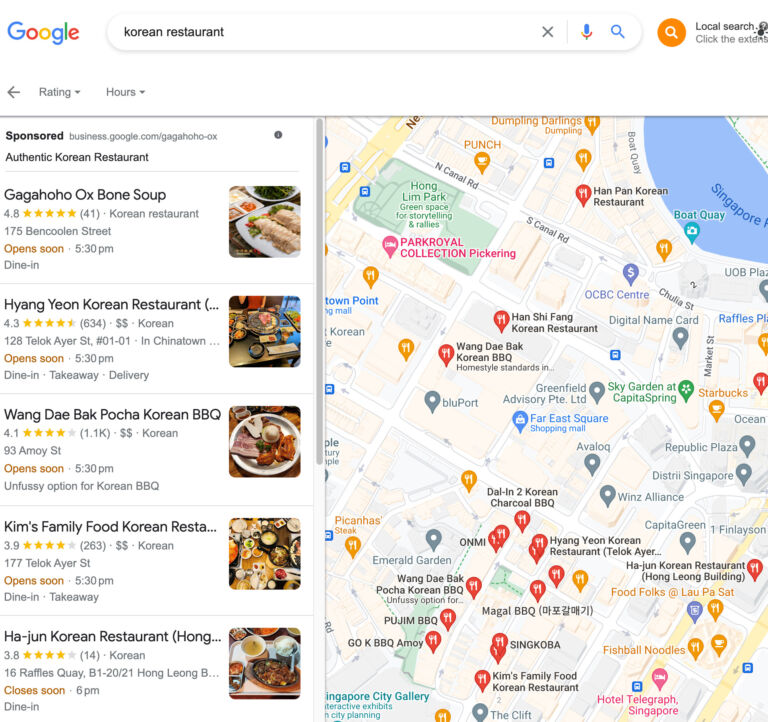The screenshot shows a Google Maps search for Korean restaurants in Singapore. On the right side of the screen, there is a map displaying various points of interest with markers in different colors: red for Korean restaurants, orange for non-Korean restaurants, and other symbols for notable locations like Boat Quay and transit spots. The top right quadrant of the map includes a body of water labeled "Singapore."

To the left of the map, there is a listing of several Korean restaurants, complete with ratings. Among them are Gagahoho, Oxbone Soup, Hyang Yeon, Hwangdae Bak Pocha, Kim's Family Food, and Ha-Joon Korean Restaurant. Notably, Hwangdae Bak Pocha stands out with over 1,000 ratings, making it one of the most reviewed spots. Him Long Park is also noted nearby on the map.

The caption for the image is: 
"Screenshot of a Google Maps search for Korean restaurants in Singapore. The map on the right highlights various Korean eateries (marked in red) alongside other points of interest, including Boat Quay and transit locations. A body of water labeled 'Singapore' is visible in the top right. The left panel lists several Korean restaurants, such as Gagahoho, Oxbone Soup, Hyang Yeon, Hwangdae Bak Pocha, Kim's Family Food, and Ha-Joon Korean Restaurant, each accompanied by user ratings. Hwangdae Bak Pocha is particularly notable with over 1,000 reviews. Him Long Park is also indicated nearby on the map."